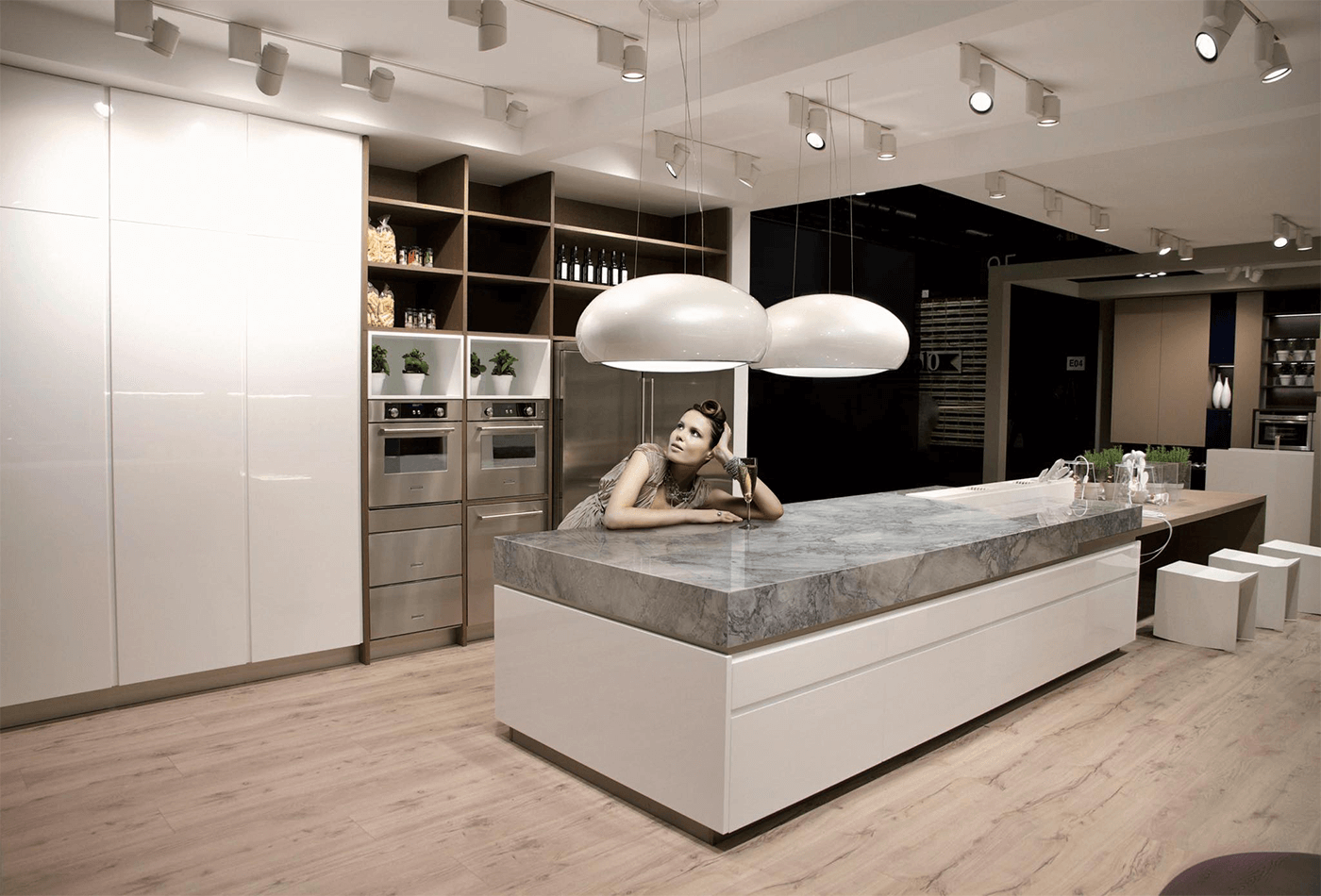In this detailed kitchen scene, a woman with curled brown hair, dressed in a gray and brown dress, is posing while leaning on a polished, dark gray marble countertop of a central island. Her left hand rests on her head, and her right hand touches the countertop. The island features a white base with storage and is surrounded by white box-like stools. A wine glass with a drink is in front of her. The kitchen boasts light brown hardwood floors and a ceiling with numerous spotlights. Behind her, there are double ovens, a double refrigerator with a metallic silver finish, and additional cabinetry of both sleek white panels and warm wooden units. A built-in table and long stools are also seen. To the left, there are shiny white panels on the wall, and the right side reveals wood elements and additional plants, including a dark wooden shelf adorned with bottles and white pottery. The overall setting of the kitchen is modern and spacious.